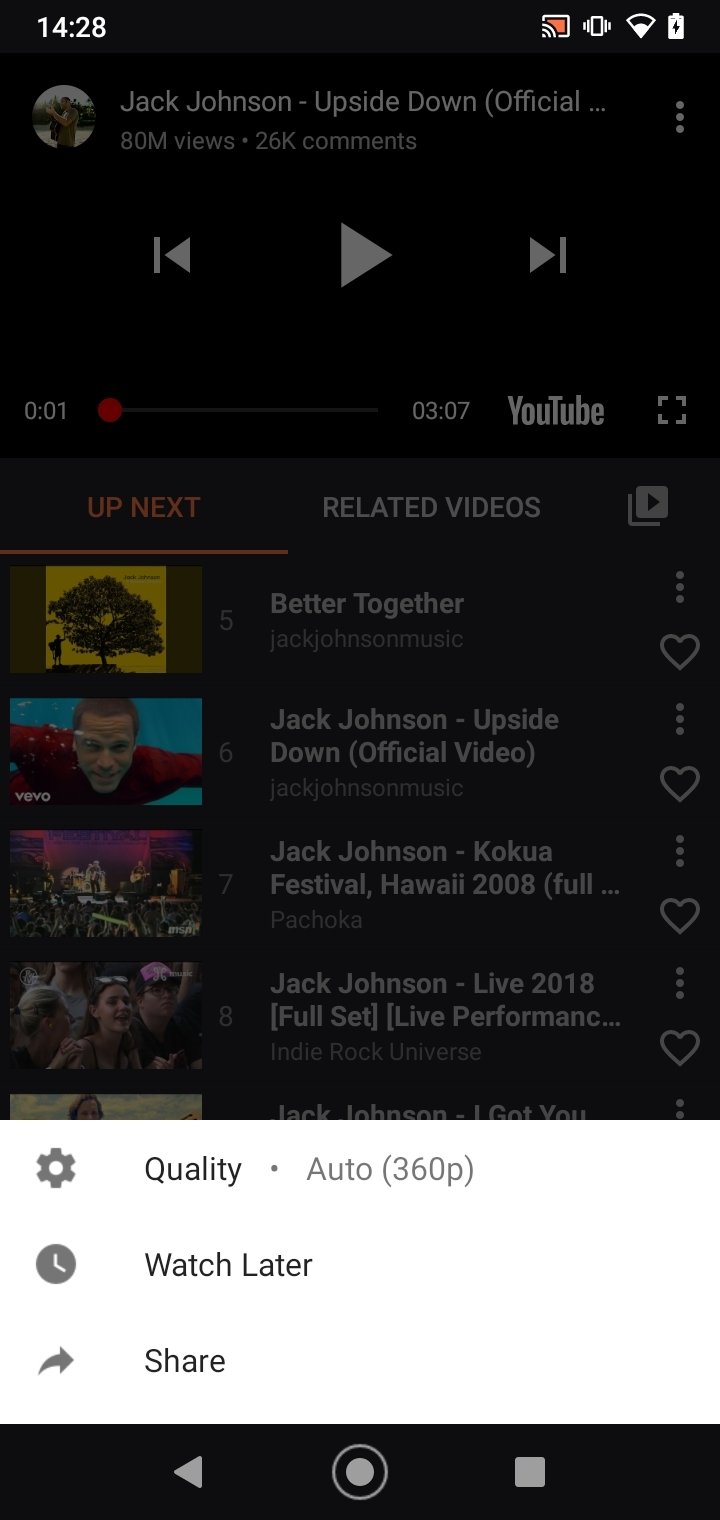The image captures a screenshot from a phone displaying a YouTube video interface. The phone's battery indicator is in the red, indicating low battery life. The time shown is 14:28. The video is titled "Jack Johnson - Upside Down (Official…)" with over 80 million views and 26,000 comments. The screen shows the standard YouTube playback controls: play, rewind, and fast forward, with the video currently paused at 0:01, indicated by a small red dot on the progress bar.

At the bottom of the screen, there's a white rectangle, making the background appear darker. This rectangle contains the options "Quality: Auto" with "360P" indicated in parentheses, a "Watch Later" button, and a share arrow symbol. Above this, the section titled "Up next" lists related videos including "Better Together," "Jack Johnson - Upside Down," "Jack Johnson Kaikou Festival, Hawaii 2008," and "Jack Johnson Live 2018 Full Set Live Performance."